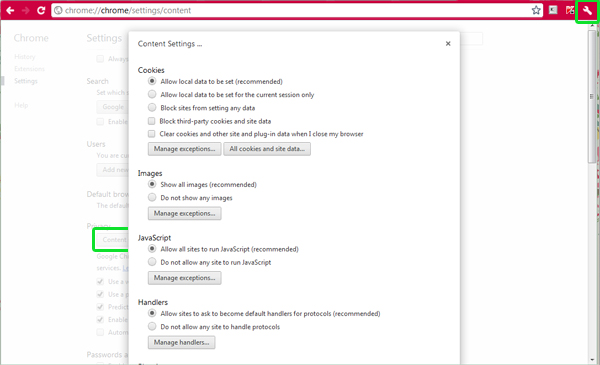The image is a detailed screenshot of the Google Chrome browser’s settings page, showcasing the comprehensive content settings section. The browser itself features a striking shade of red, almost magenta, with a long white address bar displaying "chrome://settings/content" in gray text.

In the highlighted settings section, the top heading reads "Content settings." The first category is "Cookies," with the pre-selected option "Allow local data to be set (recommended)." Additional options include "Block third-party cookies and data," "Block sites from setting any data," "Allow local data to be set for the current session only," and "Clear cookies and other site and plugin data when I close my browser." Below these options, there are two gray buttons labeled "Manage exceptions" and "All cookies and site data."

Following the cookies settings, the next category is "Images," with "Show all images (recommended)" as the selected option. The alternative option is "Do not show any images," followed by a gray button for "Manage exceptions."

Next, the "JavaScript" section offers the recommended choice, "Allow all sites to run JavaScript," with an alternative "Do not allow any site to run JavaScript" option. A gray "Manage exceptions" button is also present here.

The final category, "Handlers," includes the recommended setting to "Allow sites to ask to become default handlers for protocols" and the alternative "Do not allow any site to handle protocols." This section also includes a "Manage exceptions" button.

The background of the entire settings page is white, providing a clean and clear contrast to the gray text and options, ensuring all settings are easily readable.